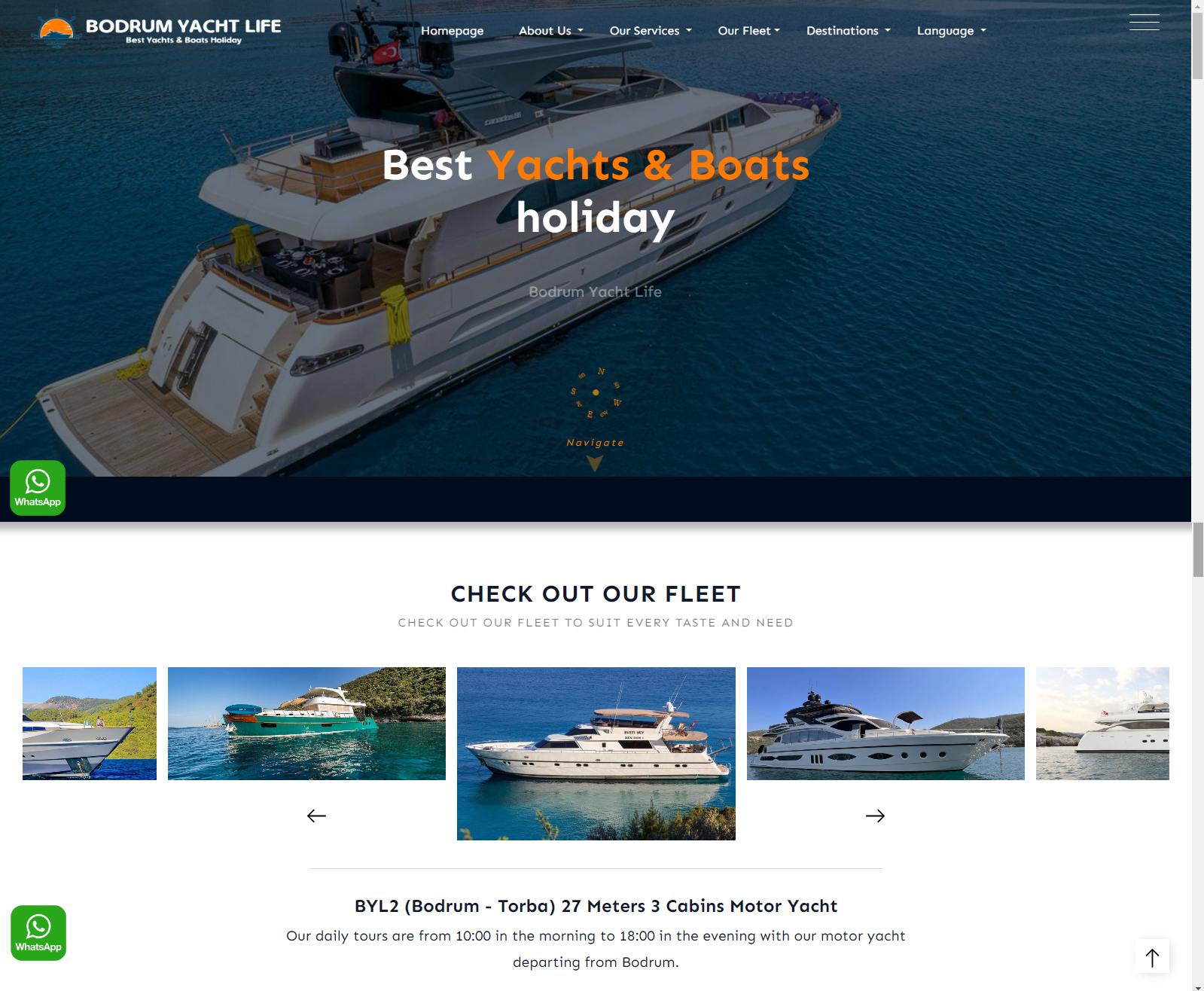Landing Page of Bodrum Yacht Life: Experience the Best Yachts and Boats Holiday

The landing page for Bodrum Yacht Life features a clean and inviting design, dominated by a captivating image of a sleek, white, two-level yacht gliding serenely on the water. This small yacht, suitable for 2-6 people, is the central visual element against a serene, unobstructed water backdrop. At the very top of the screen, the navigation menu displays categories including Homepage, About Us, Our Services, Our Fleet, Destinations, and Language options, providing easy access to various sections of the website.

Below the striking yacht image, a bold headline declares "Best Yachts and Boats Holiday," emphasizing the company's commitment to exceptional maritime experiences. Accompanying this headline is a prompt to "Check out our fleet," inviting visitors to explore a diverse range of yachts tailored to suit every taste and need.

Continuing down the page, a horizontal menu showcases numerous yachts available for rental. Although the menu cuts off the leftmost and rightmost yachts due to its scrollable design, five distinct yachts are visible, spanning from compact, personal vessels to larger options accommodating bigger groups.

Highlighted prominently below the main yacht image is a specific tour offering: "BYL to Bodrum Tour," featuring a 27-meter motor yacht with 3 cabins. Descriptive text provides further details, noting that "Our daily tours are from 10:00 AM to 6:00 PM, departing from Bodrum," conveying essential information about the tour schedule.

Overall, the Bodrum Yacht Life landing page effectively communicates the luxurious and personal nature of their yacht rental services, promising a memorable holiday experience on the water.